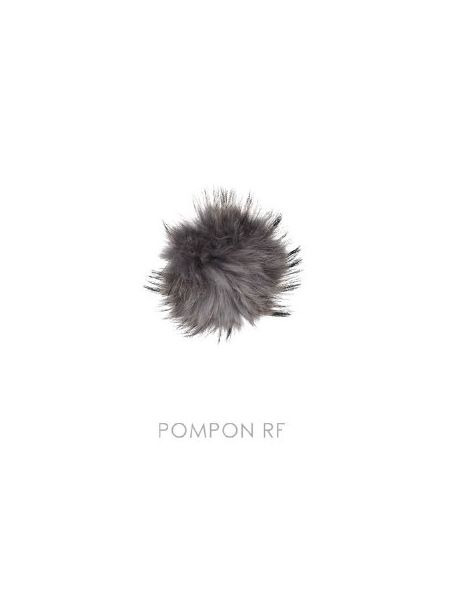The image depicts a small, furry, round pom-pom situated at the center of a plain white background. The pom-pom, resembling a dense puffball you might find on a winter hat, is primarily gray with various shades and strands of fur extending outwards in all directions. The texture appears very soft, with fur reminiscent of rabbit fur in light and medium gray tones. Below the pom-pom, there is text in a very slim, light gray font that reads "POMPON RF" in uppercase letters. The scene is minimalistic, with no other objects or people visible, drawing focus entirely to the pom-pom and the text beneath it.